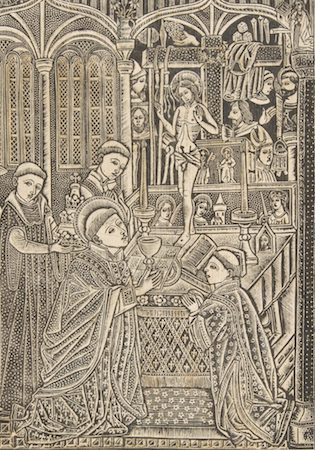The illustration depicts a detailed black and white religious scene set within a cathedral, featuring kneeling and standing monks adorned in varying patterned robes, some with crosses, dots, and diamonds. The monks, identifiable by their distinct tonsures, are gathered around an altar adorned with scripture books, candles, and goblets, engaged in what appears to be a solemn ritual or prayer. One monk on the left holds a goblet, extending it towards another monk with hands clasped in prayer. Above this interaction, a vividly drawn figure of Jesus, clothed only in a loincloth and displaying wounds on his palms, stands before the cross with his hands raised. The background is rich with detail, including numerous figures in traditional attire, such as crowns, hats, and striped head robes, enhancing the scene’s historical and contemplative ambiance. The setting is illuminated by light streaming through stained glass windows, casting a reverent glow over the tableau, with a bundle of grapes held by an unseen hand above adding to the symbolic depth of the illustration.